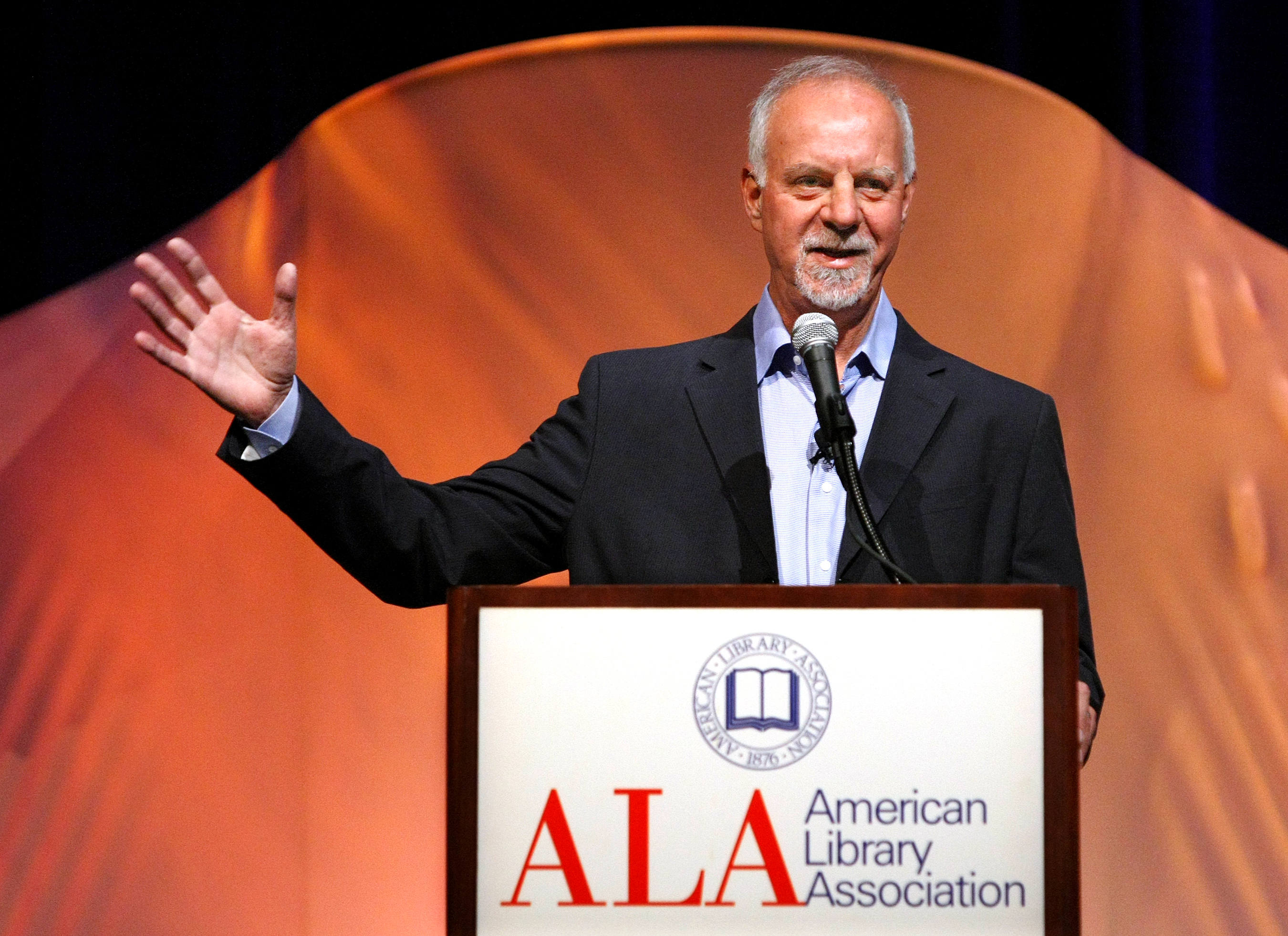In the photograph, an elderly man stands at the center of the image, delivering a speech at a podium. The background features an abstract orange-red design, which resembles a decorative seashell or a bell curve with tall sides, set against a black backdrop. The man, with grayish-white, neatly parted hair and a matching goatee, wears a black suit paired with a light blue button-down shirt, notably unbuttoned at the collar, and no tie. 

The podium displays a white sign with the red acronym "ALA" prominently, flanked by three lines of text reading "American Library Association" in black font. Above this lettering, a blue, circular emblem features "American Library Association 1876" encircling an open book. The man holds a microphone close to his face, with his right arm bent at the elbow, palm inward, while his left arm rests on the podium. The setting suggests an indoor venue, likely during an official speech.